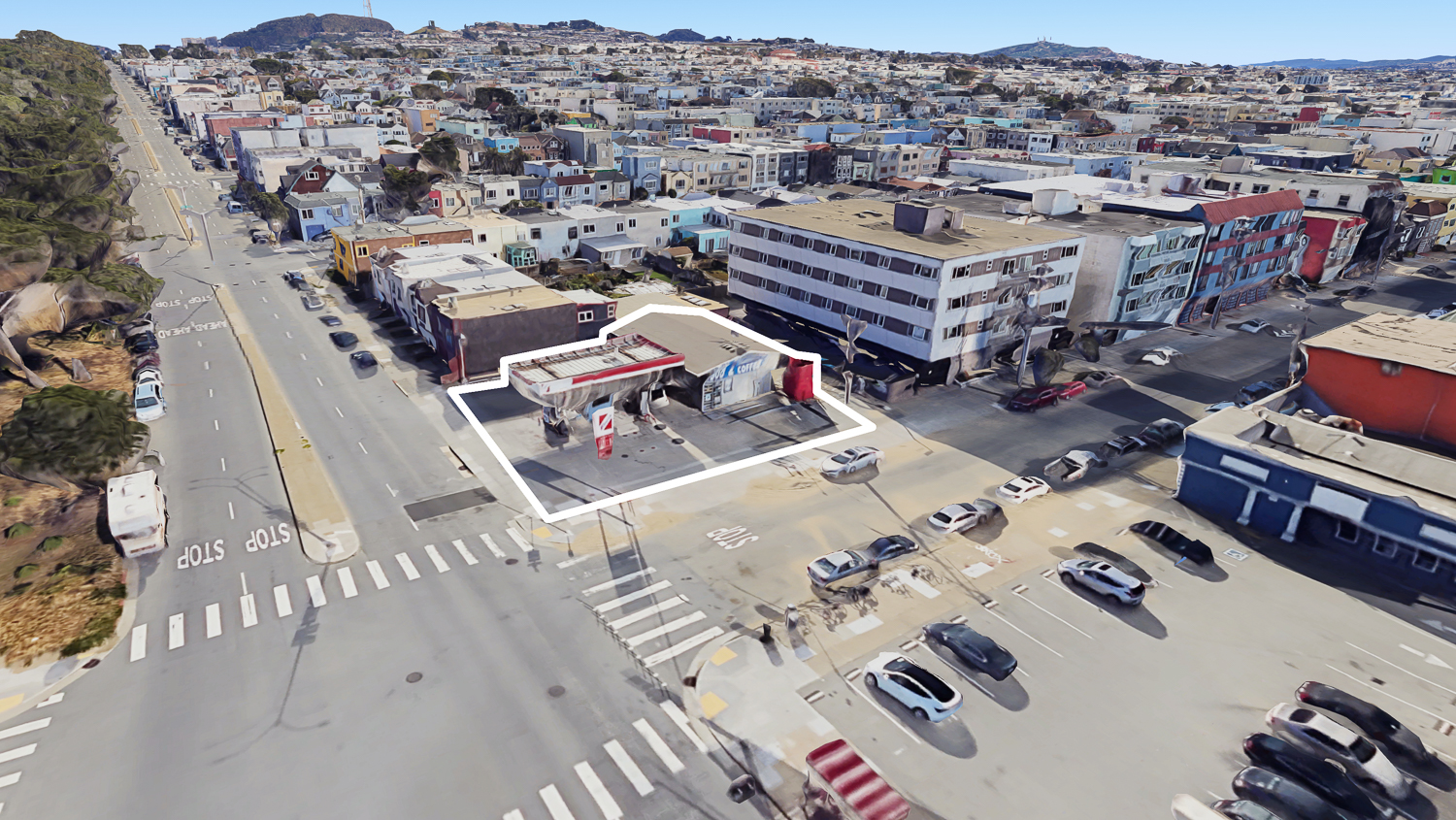This aerial photo, likely taken by a drone or a high-mounted camera, captures an extensive view of a densely populated urban area. The cityscape is crowded with a variety of tall, flat-roofed buildings in different colors, some of which appear heavily damaged, possibly due to a recent hurricane or tornado. Roofs are missing, walls are partially collapsed, and many structures are in a state of disrepair. Amidst the urban sprawl, certain buildings, such as a highlighted convenience store or gas station, stand out with clear white outlines. The image spans from a packed parking lot filled with cars at the bottom right, to the bustling city streets with noticeable details like a paved road, a white crosswalk, and a stop sign in English. In the background, a body of water suggests the presence of an ocean, while the left edge of the photo transitions from the dense city to verdant mountains dotted with greenery and dirt. The photograph also captures a portion of the blue sky, providing a stark contrast to the destruction below. The scene, possibly from the Middle East, vividly portrays a busy, yet battered, urban environment under a calm sky.